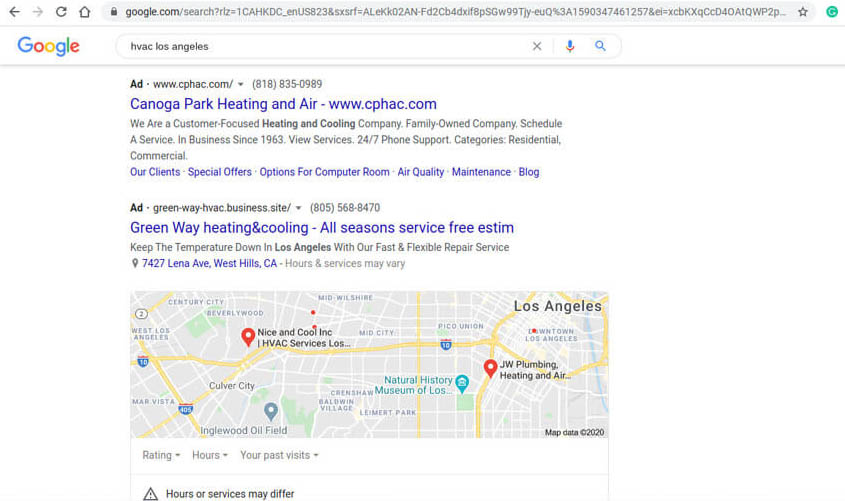This screenshot captures a desktop browser displaying a Google search result for the query "HVAC Los Angeles." The image predominantly features a white background with black, gray, and blue text. At the top, the browser URL is visible. Below that, on the left side, the Google logo is displayed adjacent to the search bar containing the entered search term "HVAC Los Angeles."

The initial two listings in the search results are advertisements, highlighted with blue headlines. The first ad headline reads "Canoga Park Heating and Air" with the URL "www.cphac.com." The second ad features "Greenway Heating and Cooling" with the subtext "All Seasons Service Free Estimate."

Directly below the advertisements, there is a map of the Los Angeles area. The map features red markers representing different HVAC service providers. The left marker indicates "Nice and Cool Ink HVAC Services Los Angeles," while the right marker points to "JW Plumbing Heating and Air Conditioning." Additional red dots mark other search results, though they are not labeled with names. The Natural History Museum of Los Angeles is also identified on the map, serving as a landmark reference.